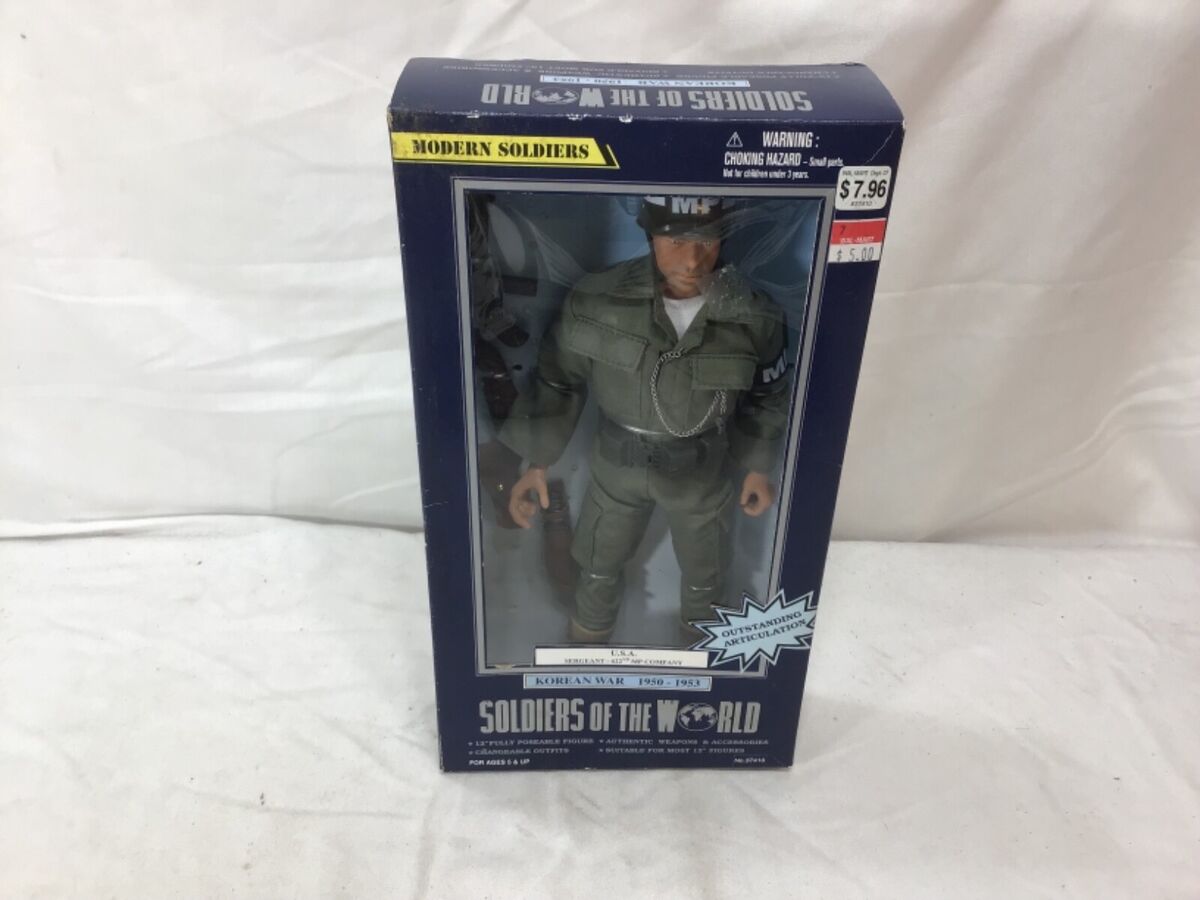The photograph features a toy soldier action figure encased in a dark navy blue box, placed on a white drape background. The front of the box prominently displays the words "Modern Soldiers." At the top and bottom of the box, it reads "Soldiers of the World, Korean War, 1950-1953," though the text at the top is upside down. The box incorporates a see-through rectangular window, showcasing the action figure inside, who is dressed in green military fatigues with a hat marked "MP." The figure, with fair skin, stands in a neutral position and expression, surrounded by various accessories including a small black gun. On the right side of the box are two price stickers: a $7.96 sticker and an older Walmart sticker priced at $5.00.